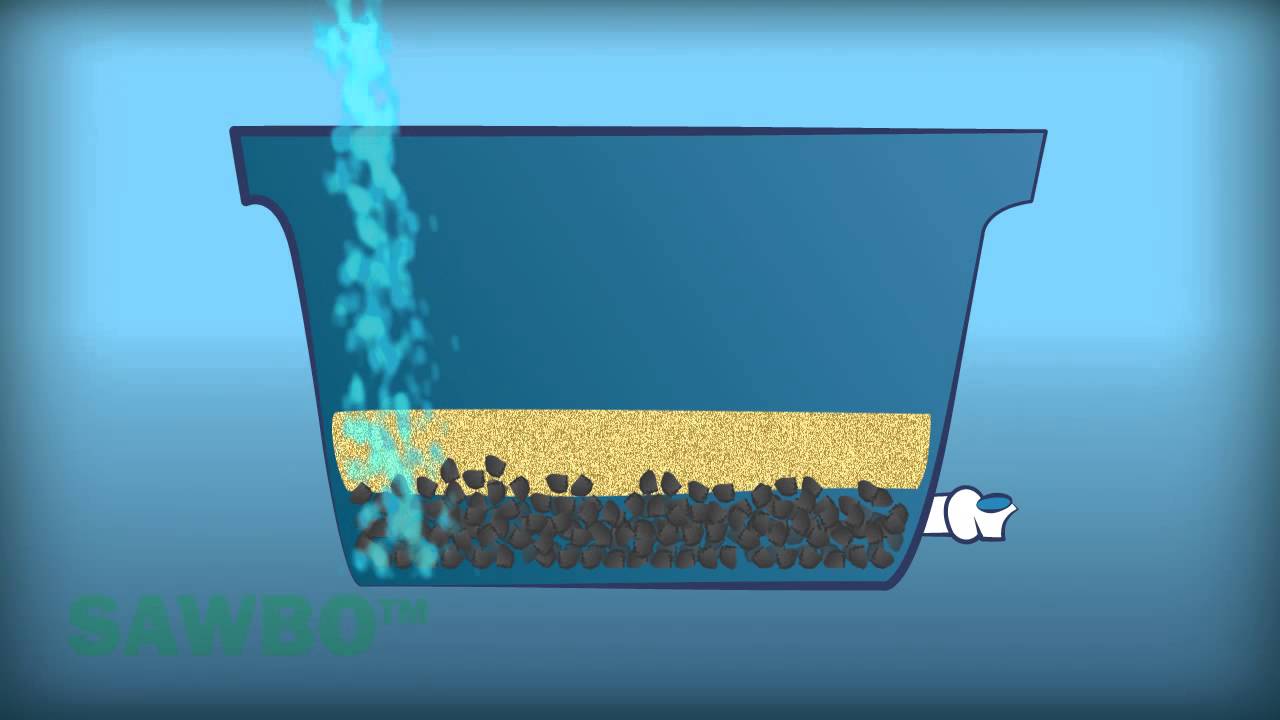The image features a blue container or pot set against a blue background that transitions from a lighter blue at the top and middle to a darker blue towards the bottom. The container itself appears to be a digital drawing and is centrally placed within the composition. Emanating from the left side of the container is steam, depicted in shades of white and blue. The design of the container includes lips on both ends with rounded edges at the bottom.

Towards the bottom of the container, there is a layered section. The first layer above the bottom consists of a tan filter, resembling cork or a band-aid with small, precise dots. Beneath this, there is a layer of small, round black dots that look like charcoal bits or coffee beans. At the very bottom of the container, aligning with these black dots, is a small white spout with a blue circle or button on top, likely serving as an outlet for the contents of the container.

Additionally, on the left side of the image, there is some green, semi-transparent writing that appears to say "S-A-W-B-O-T-M," though it blends into the background and is difficult to decipher. The overall aesthetic of the image combines elements of both solid fill and detailed patterning against the blue gradients of the background.